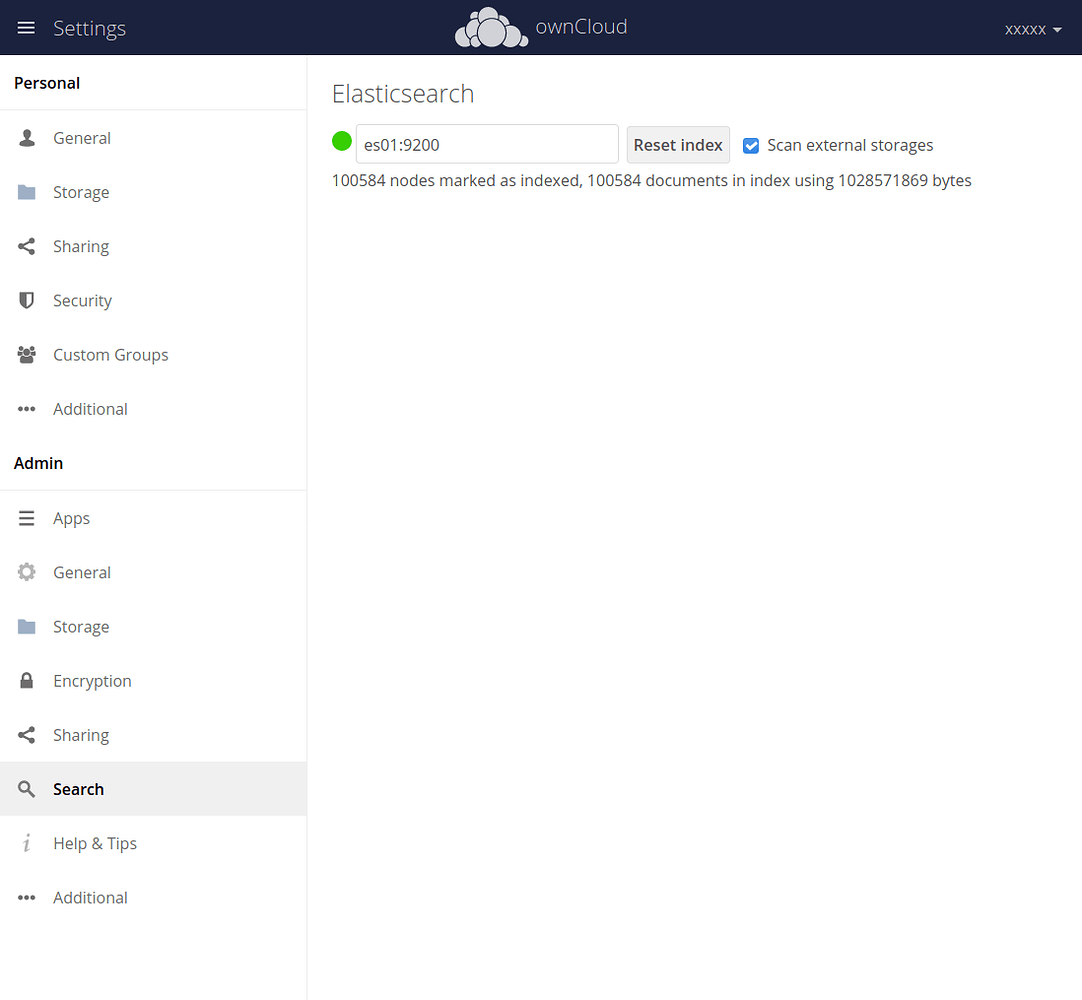Here is a more polished and detailed caption for the image you described:

---

The image displays a settings profile screen within an app. In the upper left corner, there is a white three-line options button next to the word "Settings." The top section of the screen, which has a blue border, features a pattern of variously sized circles clustered together, resembling a cloud with the text "Own Cloud" superimposed on it. To the far right of this section, there is a label marked "XXXXX" next to a dropdown menu. 

Below the blue-bordered area, the main part of the screen has a white background. It is segmented into several tabs for navigation: "Personal," "General," "Storage," "Sharing," "Security," "Custom Groups," and "Additional." 

When switched to the "Admin" mode, the tabs change to: "Apps," "General," "Storage," "Encryption," "Sharing," "Search," "Help and Tips," and "Additional." The "Search" tab is specifically highlighted, showing detailed search settings. Below the "Search" heading, it is labeled "Elastic Search" with an accompanying search box displaying "ES01, 9200." There is also a checkbox for "Reset Index Scan Internal Storages," which is checked. Additional information indicated that there are 100,584 nodes marked as indexed and 100,584 documents in the index, utilizing 1,028,571,869 bytes of storage.

---

This caption provides a comprehensive and detailed description of the image, giving a clear understanding of the layout and the specific elements present in the settings profile screen.